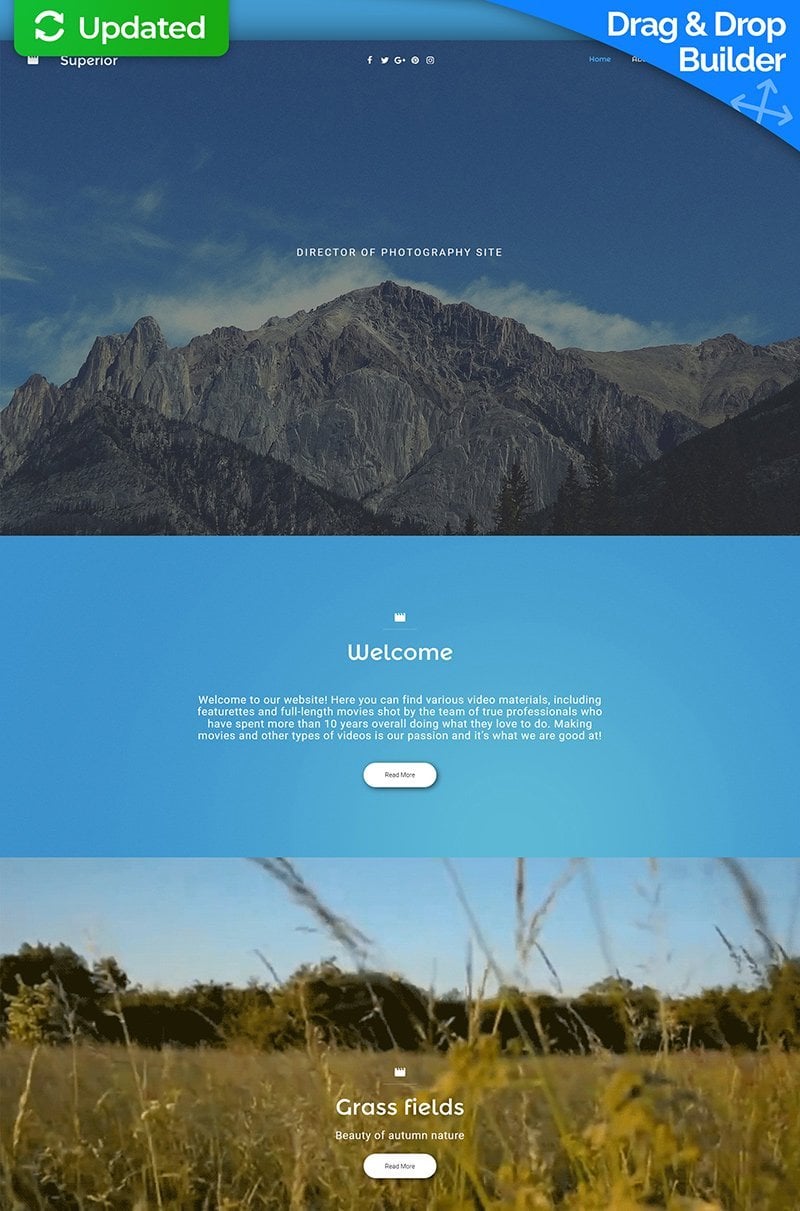The image features a screenshot of a minimalist website builder interface. In the upper left corner, there is a green button with the white text "Updated." On the upper right, a triangular-shaped banner with a blue background and white text reads "Drag-and-Drop Builder." The interface appears user-friendly, allowing users to click on different sections to edit text and other elements easily. The first section showcases a picture of a mountain, while the second section features a gradient blue background transitioning from rich sky blue to a greenish-blue in the center. The final section displays a serene image of grass fields accompanied by the words "Grass Fields" in white text and a "Read More" button.